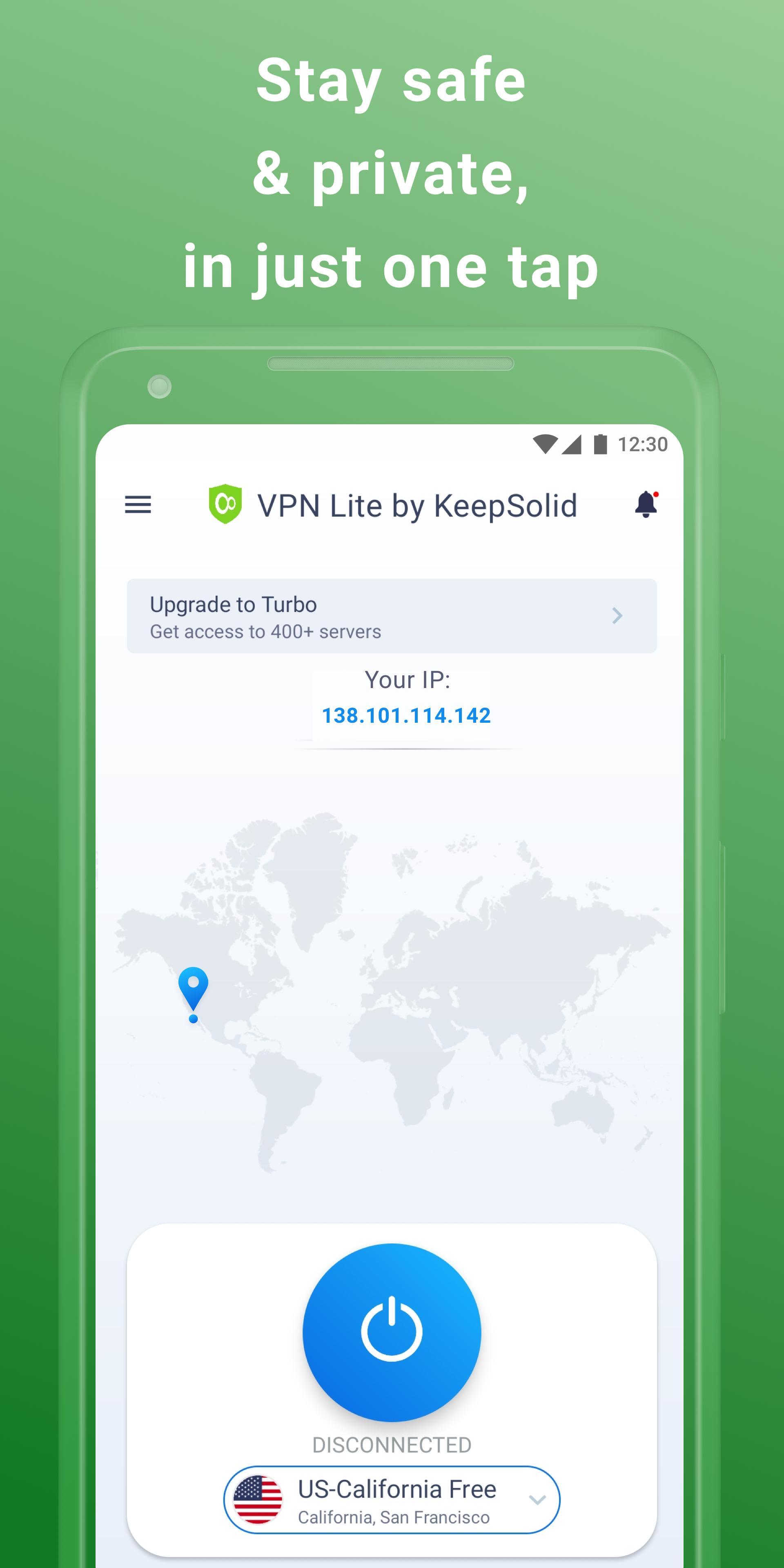The image is an advertisement with a green gradient background that features prominent white text saying, "Stay Safe and Private in Just One Tap." Overlaid on the background is an outline of a generic smartphone, possibly an Android, with a fully opaque screen displaying all its details clearly. 

On the screen's taskbar, the time is displayed as 12:30, located on the top right. The top left corner shows the application name, "VPN Lite by Keep Solid," accompanied by a three-line menu button. On the opposite side, a black bell icon signifies notifications or alerts.

Below the taskbar, a world map is displayed with text encouraging users to "Upgrade to Turbo" to gain access to over 4000 servers. A specific IP address, 138.101.114.142, is shown, with a map pin indicating a location likely in California.

At the bottom of the screen, there is a blue "Off" button with a white symbol, showing the VPN status as "Disconnected." Below that, a dropdown menu features a small avatar with an American flag icon, listing the connection as "U.S., California free, California, San Francisco," confirming the location marked by the pin on the map.